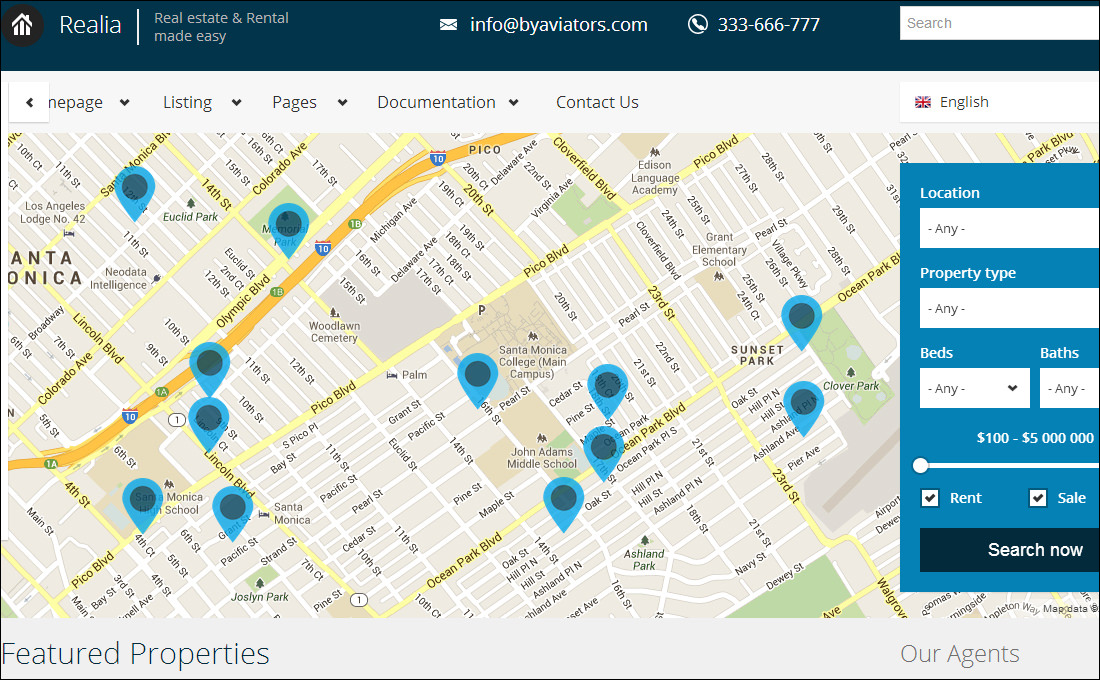This screenshot from a real estate website features a comprehensive interface designed to streamline the process of finding rental and sale properties. At the top of the page, a navigation bar displays a house icon followed by the text "Relia," which stands for Real Estate and Rental Made Easy. Adjacent to it is an envelope icon with the email address "info@buyaviators.com" and a telephone icon showcasing the number "333-666-777." Note that the phone number appears incomplete as it lacks one digit.

The navigation bar also includes a search field labeled "search." Alongside the search field, headers read "Listing," "Pages," "Documentation," and "Contact Us," albeit one header is partially cut off. On the far right, a British flag icon accompanied by the word "English" indicates the selected language is British English.

A prominent map dominates the page, marked with numerous pins that likely denote available real estate properties in an area that seems to be around Santa Monica, as the word "Santa" is partially visible. Nestled on the right side of the map, there is a filtering box allowing users to refine their property search. Filter options include "Location," "Property Type," "Beds," and "Baths," each preset to "Any" but adjustable via dropdown menus. A price range slider stretches from $100 to $5 million, and two checkboxes for "Rent" and "Sale" are selected, implying the search encompasses both rental and sale properties.

At the bottom of the screenshot, sections labeled "Featured Properties" and "Our Agents" suggest additional functionalities providing further insights and support.

Overall, the website's layout is intuitively designed to facilitate easy browsing and filtering of real estate listings, offering a user-friendly approach to finding desirable properties.